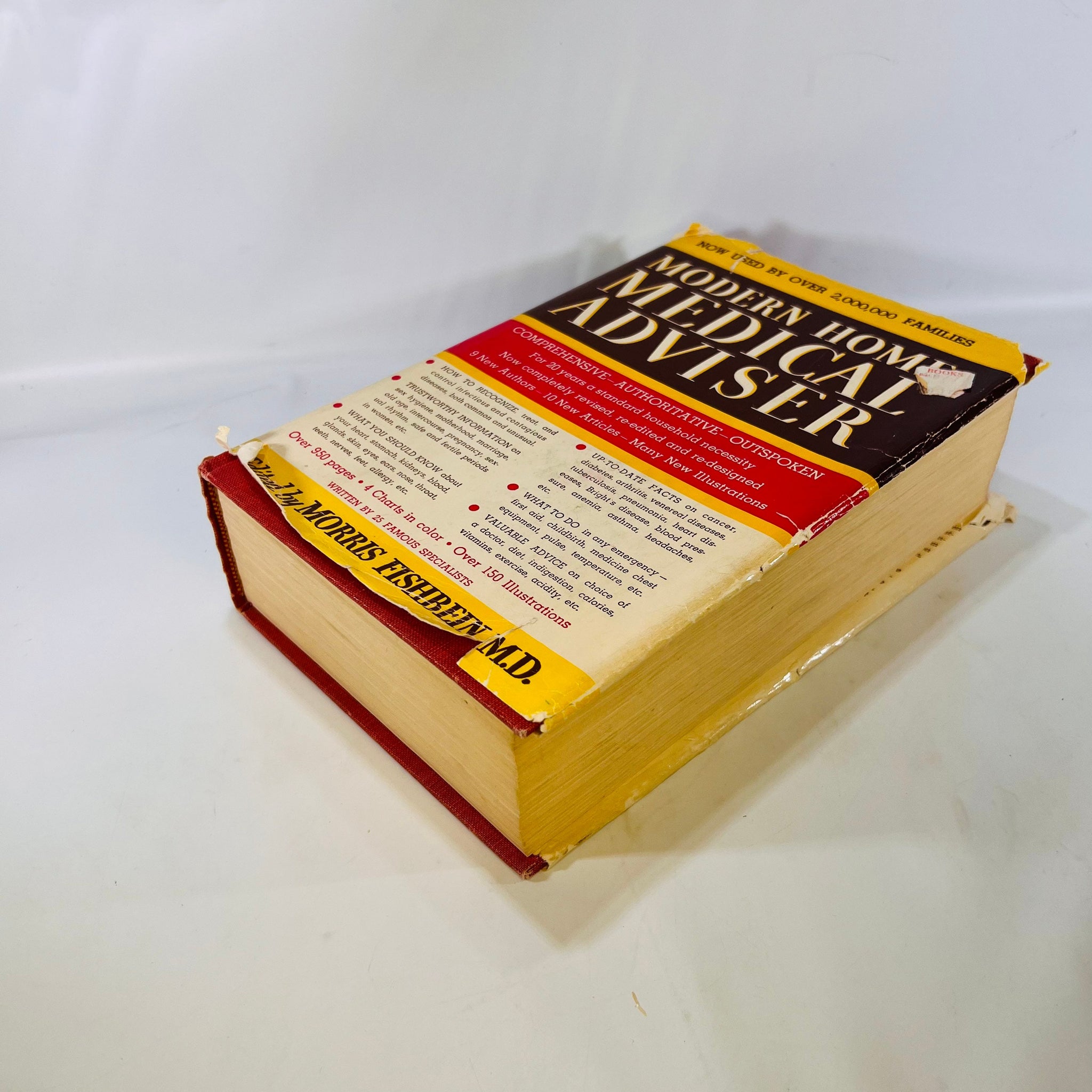The image depicts a well-worn and heavily damaged copy of "Modern Home Medical Advisor" by Morris Fishbein, MD. The book is set against a white background, which is partially obscured by slight shadows. The book's jacket is primarily composed of black, red, yellow, and white banners, with white text on a black banner prominently displaying the title. Below the title, a red banner framed in gold continues with additional information. The cover is significantly damaged, particularly at the bottom where it is ripped in two places, and a portion of the cover where the 'E' in "HOME" is located is missing. The bottom section of the cover includes text asserting, "Now used by over two million families," along with the author's name. The front cover also offers valuable advice and facts by the medical advisor. The pages of the book are yellowed with age and show signs of wear. Beneath the tattered jacket, the book itself is red, with more wear and slight tears visible on the lower part of the jacket.